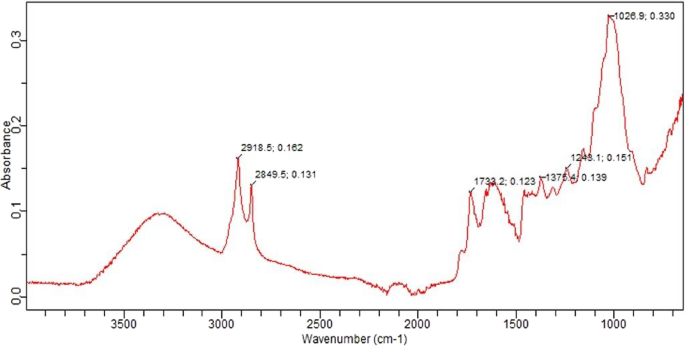This image is a detailed scan of a line chart illustrating absorbance versus wave number (cm⁻¹). The x-axis, labeled as "wave number (cm⁻¹)", features major tick marks at 3500, 3000, 2500, 2000, 1500, and 1000. The y-axis, labeled "absorbance", is marked at intervals of 0.0, 0.1, 0.2, and 0.3. 

A red line begins around the y-value of 0.002 and runs horizontally before rising to a local maximum of approximately 0.01 near the 3400-3300 cm⁻¹ range. It then descends sharply at the 3000 cm⁻¹ mark before spiking significantly at 2918.5 cm⁻¹ and 0.162 absorbance. The line dips again and rises to another peak at 2849.5 cm⁻¹ and 0.131 absorbance before exhibiting further peaks and valleys.

Notable points of the line include a rise to about 0.01 absorbance at 1732 cm⁻¹, then downwards, and up to 0.139 absorbance at 1374 cm⁻¹. The line continuously oscillates, and near 1026 cm⁻¹, it peaks at 0.33 absorbance before slightly dropping and eventually rising above 0.2 absorbance towards the lower end of the spectrum. Key labeled points include 2918.5 cm⁻¹, 0.162 absorbance, and 2849.5 cm⁻¹, 0.131 absorbance among others.

Overall, this line chart meticulously maps the absorbance variations across different wave numbers, highlighting significant peaks and trends in the data.